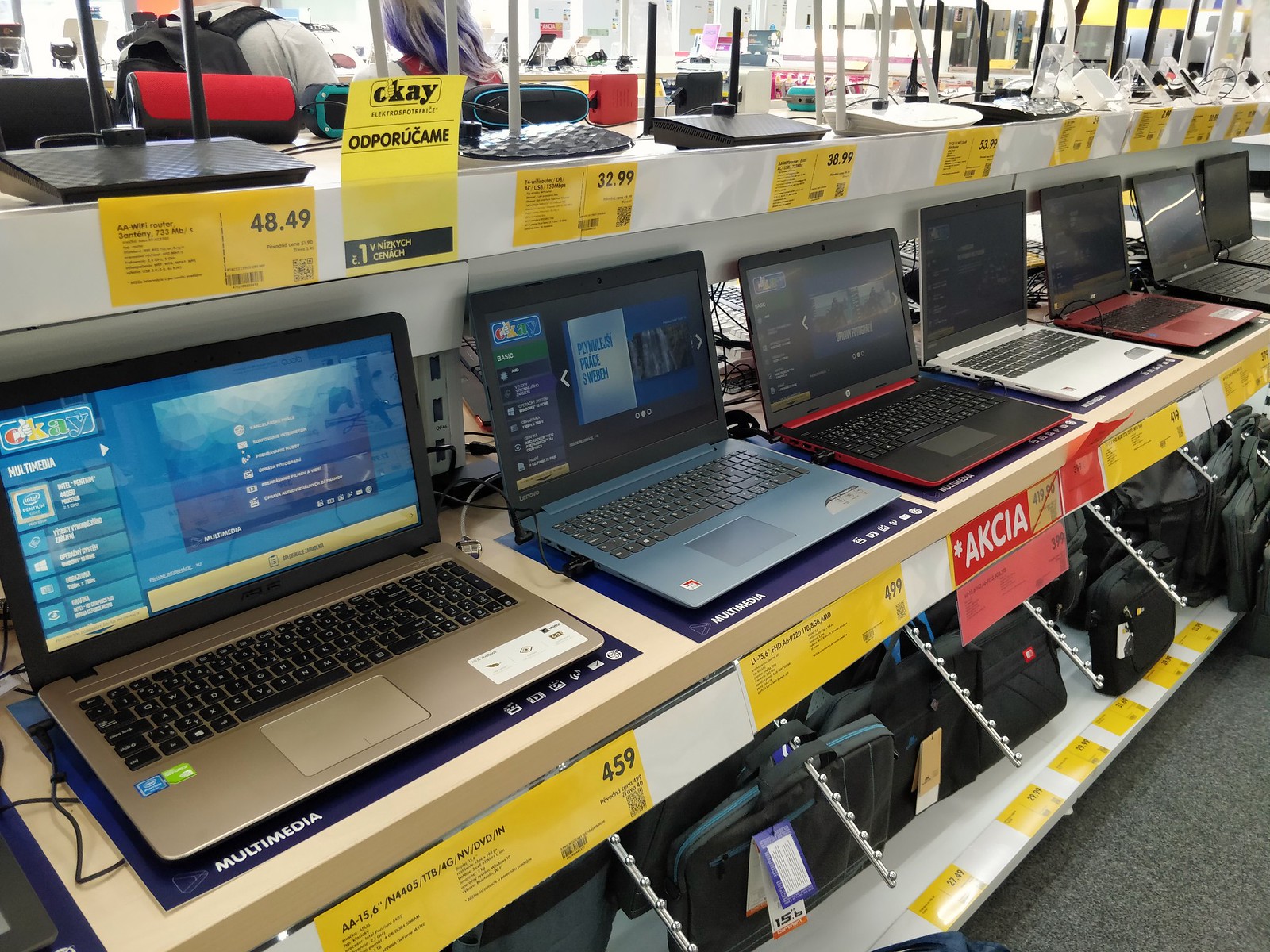Inside an electronic store similar to Best Buy, the focus of the image is a display of three shelves. The middle shelf holds seven laptops arranged diagonally from the bottom left corner to the top right. These laptops vary in brands, colors, and sizes, creating a vibrant array of reds, blues, whites, and blacks. Each laptop displays the same image on its screen and has a yellow price label underneath. The first laptop on the left is priced at $459 and boasts a silver and black finish with a 15.6-inch monitor, one terabyte storage, four gigabytes of RAM, and NV and DVD-N capabilities. As you move to the right, the laptops change in color, including blue, red, white, and black variations.

Beneath the laptops, the bottom shelf features black attache-style carrying cases for laptops, hanging from small hooks. These cases differ in sizes and brands but lack individual price labels. Above the laptops, the top shelf houses a variety of Wi-Fi routers or extenders, again varying in brands and colors. Yellow price labels are scattered throughout the display but in a language that suggests the store might be located in Eastern Europe. In the background, a couple of shoppers can be seen, their heads partially turned away from the camera, adding to the busy atmosphere of this electronic haven.